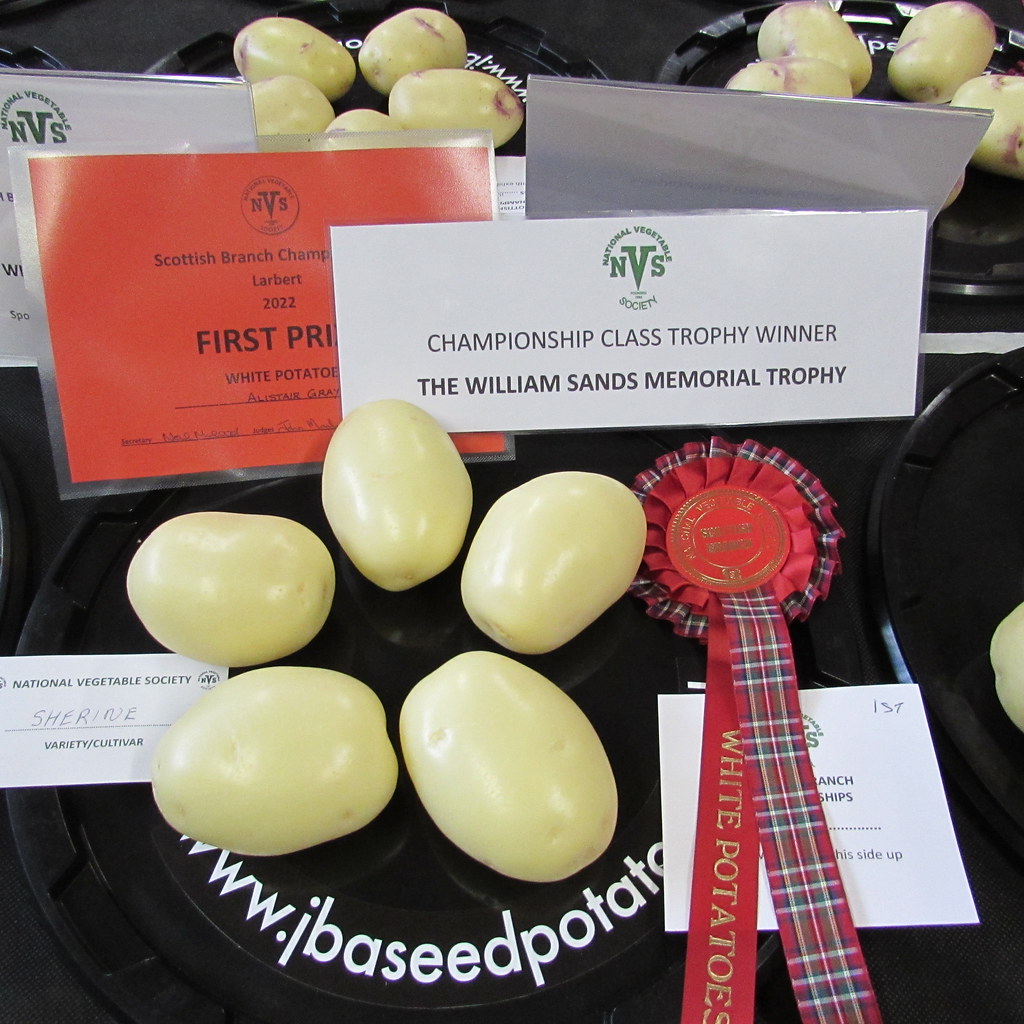The image depicts a cooking competition table featuring multiple black circular plates, each containing five potatoes. Each plate is accompanied by various award cards and ribbons. One prominent card, with a red header and the NBS (National Vegetable Society) logo, reads "Scottish Branch Championship 2022, First Prize, White Potatoes, Alistair Gray." Another card with the NBS logo states "Championship Class Trophy Winner, The William Sands Memorial Trophy." Additionally, there's a plate identified by a card reading "National Vegetable Society, Variety/Cultivar Sharing," and it includes the website www.jbaseheadpotato. A red ribbon with gold lettering that says "White Potatoes" is also notable in the arrangement. In the background, additional potatoes and related awards can be seen, emphasizing the competitive and celebratory nature of the event.